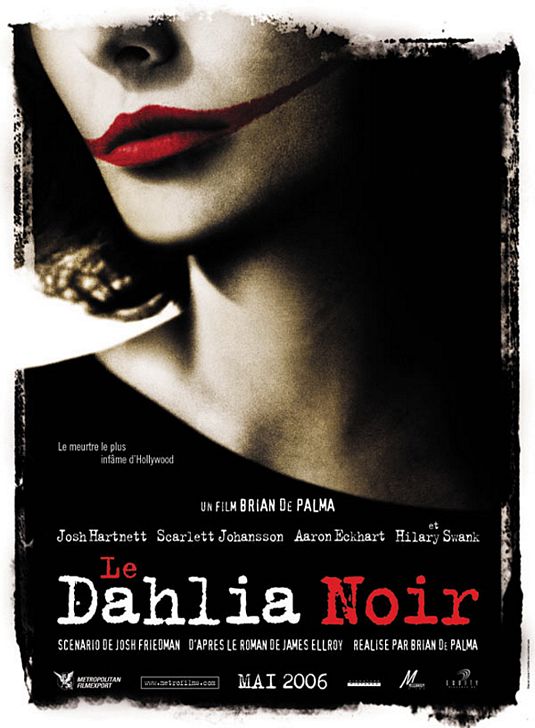The movie poster for "La Dahlia Noire" (The Black Dahlia) is a striking black-and-white image with elements of red. The focus is on the lower half of a woman's face, from her neckline to just below her nose. She has bright red lipstick that extends past her lips and smears across her cheeks, reminiscent of the Joker's makeup in Batman. The woman has a pale complexion and dark hair, complementing the noir aesthetic of the poster. The edges of the poster are deliberately distressed, mimicking torn or melted celluloid film, adding an old, vintage feel. The title "La Dahlia Noire" and the director "un film Brian De Palma" are featured prominently, along with the names of the main actors: Josh Hartnett, Scarlett Johansson, Aaron Eckhart, and Hilary Swank. The film's release date in French, "MAI 2006", and studio markings are noted at the bottom, with the text presented in a mix of typewriter and modern fonts.